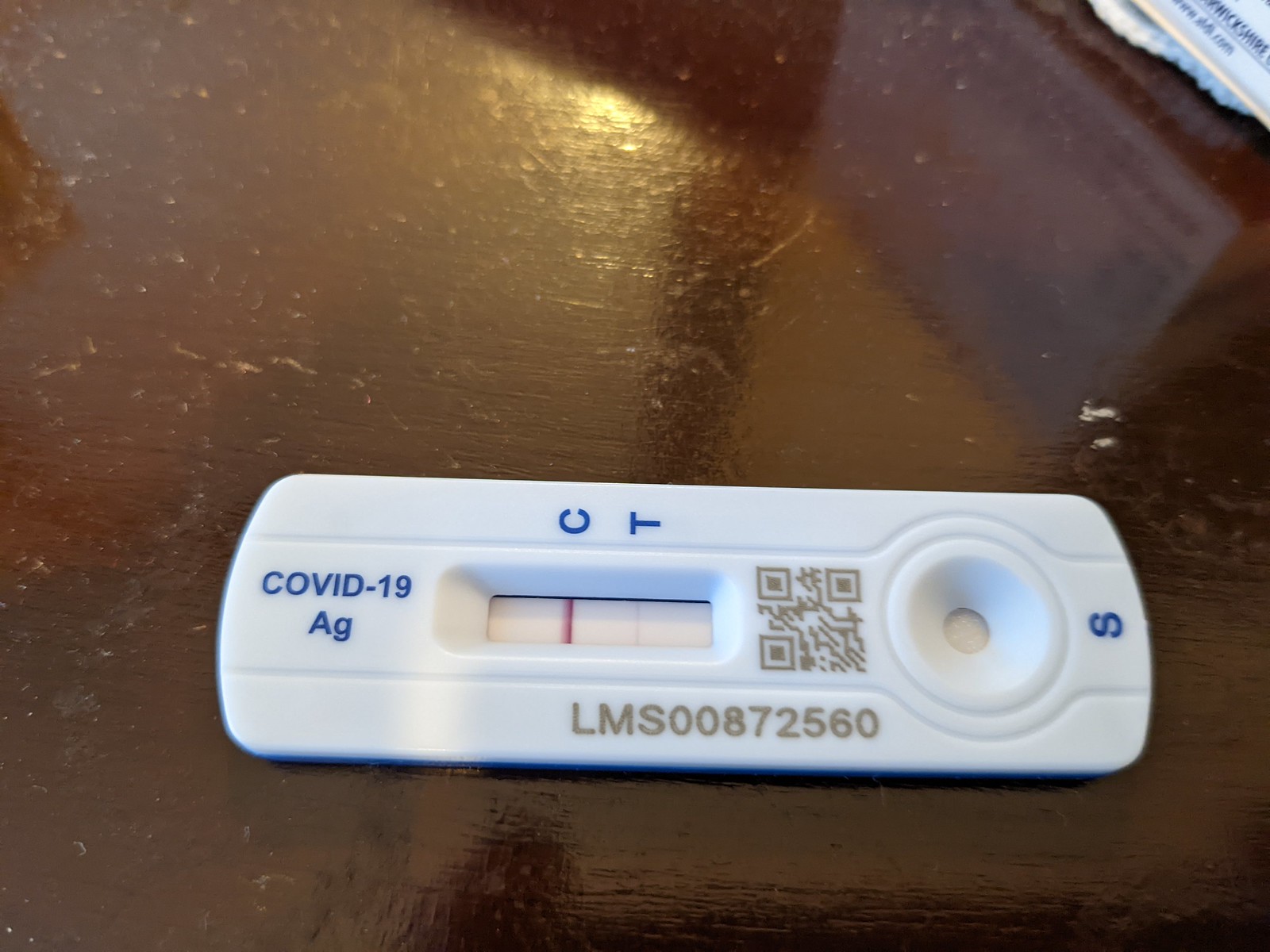The image showcases a COVID-19 test kit, prominently labeled in blue letters with "COVID-19 AG." The side of the kit features a tan-colored serial number, "LMS 00872560," and includes a QR code in the same tan hue. Positioned at the bottom is the letter "S". The test kit is viewed sideways, showing blue letters "C" and "T" along with a solid pink line near the "C". The kit is placed on a highly reflective, glossy table which mirrors the presence of a white box with blue text situated nearby. The table's surface reveals a noticeable, broad scratch and visible brush strokes in its brown paint, indicating a hand-painted finish. Additionally, a long shadow stretches across the entire image, enhancing the visual complexity of the scene.